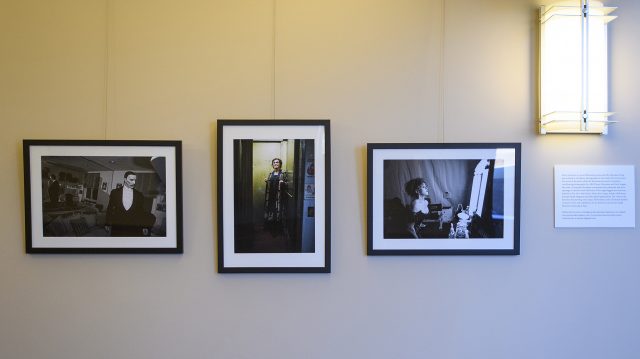The photograph captures an indoor setting, likely an art gallery or show, featuring a beige or off-white wall with three framed photographs and a white information card. The wall appears to be painted white, although the room is dimly lit, creating an overall muted color tone. The photos are arranged horizontally, each in a black frame with white matting, accompanied by a rectangular lamp in the upper right corner casting a soft, fluorescent-like white and yellow light on them. 

The photograph on the far left is a black-and-white image of a man in a tuxedo with a white tie, possibly a conductor, although the specific details of his actions remain unclear. The center image, which is in color but with minimal saturation giving it a sepia or yellowish tone, depicts a single figure, likely female, standing in a background suffused with a greenish hue. The photograph on the right, also black and white, appears to show a woman, but the details are indistinct, possibly involving a reflective surface like a mirror or window. Next to the framed photographs is a white plaque with writing that provides explanatory information, but it is too distant to be legible.